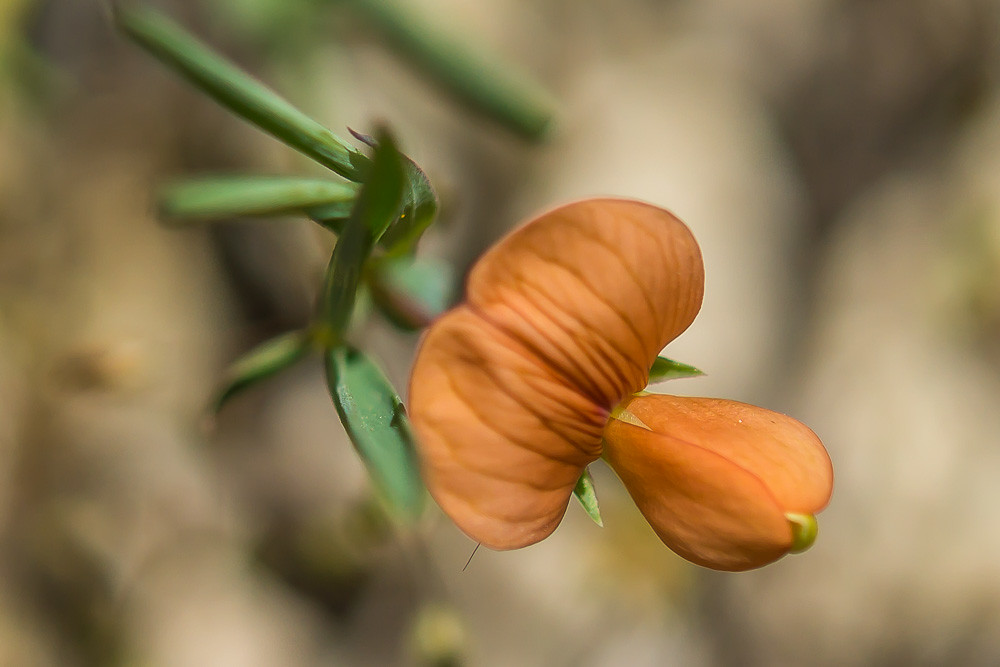The photo depicts a close-up view of an orange flower in bloom, showcasing an intricate blend of hues and textures. The flower, tinged with varied shades of orange and slight hints of yellow and brown, exhibits noticeable wrinkles, hinting at its potential age or late blooming stage. At the top of the flower bud, a small green hook-like structure is visible. The flower emerges from vibrant, green leafy stems with an earthy green coloration. Additionally, a subtle light purple hue can be glimpsed beneath the flower petals, adding depth to the image. The background is notably blurred, presenting an array of indistinct gray, black, and possibly rocky textures, emphasizing the flower's delicate details. The overall composition, wider than it is tall, maintains a sharp focus on the flower head, making it the primary subject against a muted backdrop devoid of any watermarks or extraneous objects.